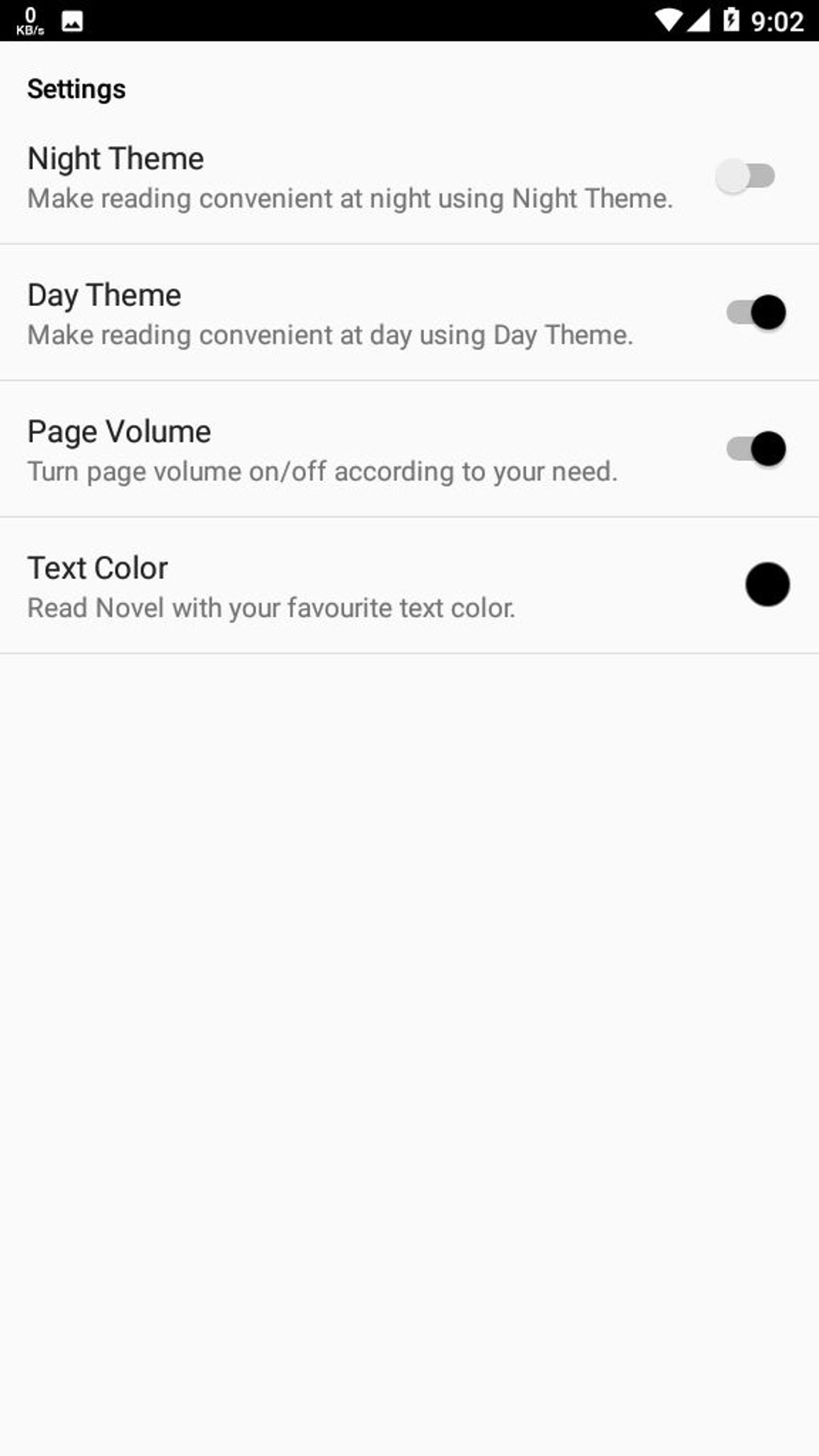The image displays a settings panel for an application or possibly for the entire phone. At the top, there is a data label showing "0 KBS per second," accompanied by an icon for a photo. The screen indicates full Wi-Fi signal, full cellular signal, and a fully charged battery, set against a clock showing 9:02. On the left side, a small header in bold text reads "Settings."

Beneath this heading, there are four options presented in larger, non-bold text:

1. **Night Theme**: 
   - Description: "Make reading convenient at night using the night theme."
   - Status: The slider for this option is set to off.

2. **Day Theme**: 
   - Description: "Make reading convenient at day using the day theme."
   - Status: The slider for this option is set to on. When on, the circle within the slider has a black dot, while in the off position, it shows a light gray dot. The slider bar itself is medium gray.

3. **Page Volume**: 
   - Description: "Turn page volume on/off according to your need."
   - Status: The slider is currently on.

4. **Text Color**: 
   - Description: "Read novel with your favorite text color."
   - Status: This option does not have an on/off slider but features a large black circle as a placeholder, perhaps representing a selectable color option.

The bottom portion of the screenshot is dominated by white space, indicating no additional options are presently visible.